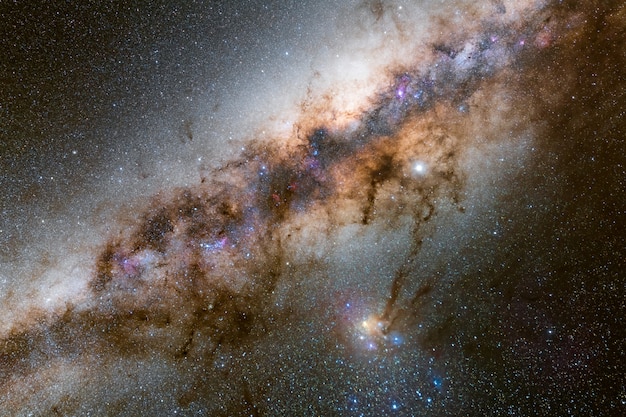An image captured through a high-powered telescope reveals a mesmerizing view of the night sky, showcasing intricate details far beyond the naked eye's reach. The background is a deep, infinite black speckled with countless bright dots representing distant stars, galaxies, or other celestial objects. Dominating the scene is a central chasm-like structure, swathed in mysterious, swirling patterns of brown, purple, and black hues. This structure is encased in a white, misty essence, lending a ghostly appearance to the cluster of stars, possibly planets, or perhaps entire galaxies it contains. The abstract formations and colors create an ominous yet captivating foreground against the dotted starry expanse, hinting at cosmic phenomena far in the depths of the universe. The presence of vibrant stars and possibly other Suns adds to the grandeur of this high-tech, space exploration photograph, depicting the captivating mysteries of outer space.